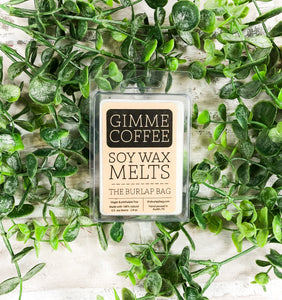The photograph, likely intended for advertising, features a small, white rectangular product prominently displayed within a transparent plastic container. The product's label reads "Gimme Coffee, Soy Wax Melts" in distinct white letters against a black and cream-colored background, with additional smaller text that is unreadable due to the image's size. The product encased in clear packaging is mounted against a white backdrop adorned with various plants, comprising vivid and light green stems and round leaves, adding a decorative touch to the composition. This thoughtfully arranged scene highlights the product's aesthetic appeal amid natural elements, enhancing its visual allure.